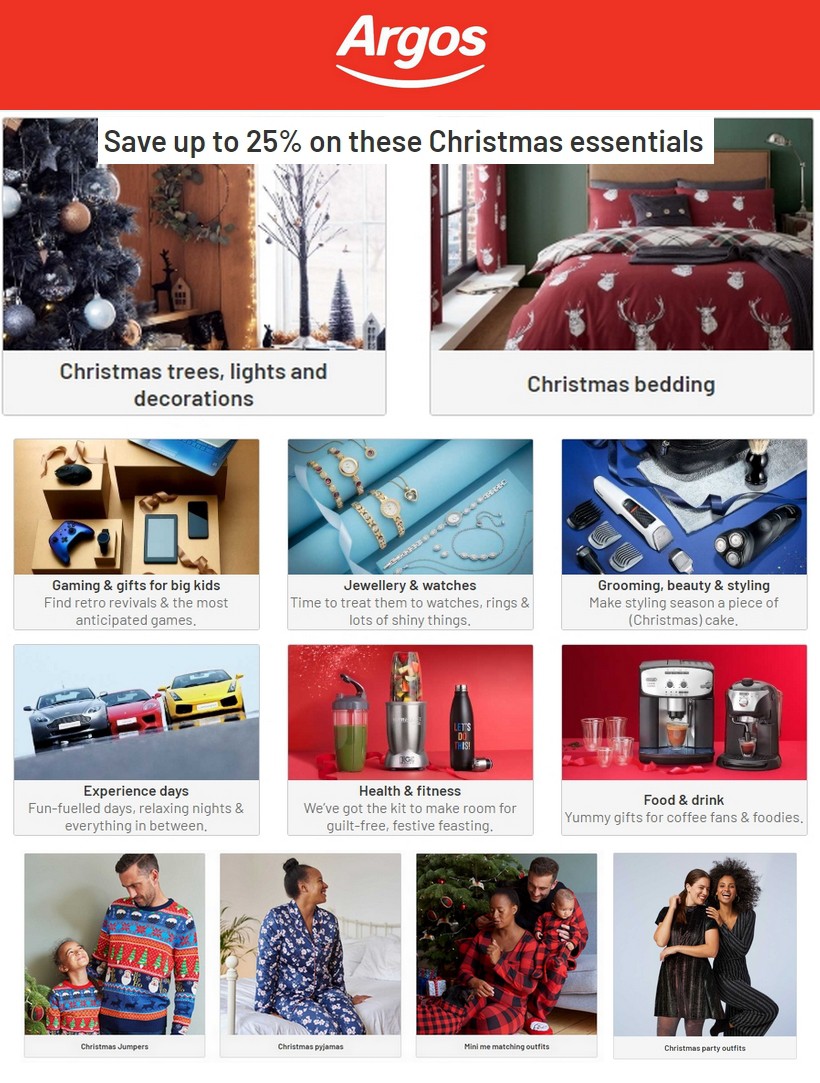Sure, here’s a clean and detailed caption for the image description provided:

---

"Screenshot of an Argos website showcasing a holiday sale. A prominent red bar at the top features the Argos logo in white, with a swoop underneath. Beneath the logo, a banner advertises 'Save up to 25% on these Christmas essentials.' The webpage is organized into several rows of boxes, each highlighting different categories of holiday items.

The first row includes:
1. 'Christmas Trees, Lights, and Decorations'
2. 'Christmas Bedding'

The second row features:
1. 'Gaming and Gifts for Big Kids'
2. 'Jewelry and Watches'
3. 'Grooming, Beauty, and Styling'

The third row highlights:
1. 'Experience Days'
2. 'Health and Fitness'
3. 'Food and Drink'

The final row presents images of people modeling holiday-themed clothing. 
1. 'Christmas Jumpers' shows a man and his daughter in matching Christmas sweaters.
2. 'Christmas Pajamas' features a black woman sitting on a bed in blue and white pajamas.
3. 'Mini Me Matching Outfits' depicts a family—comprising a black woman, a white man, and a baby—wearing matching pajamas next to a Christmas tree.
4. 'Christmas Party Outfits' showcases two women dressed up for a festive occasion."

---

Let me know if you need further assistance!